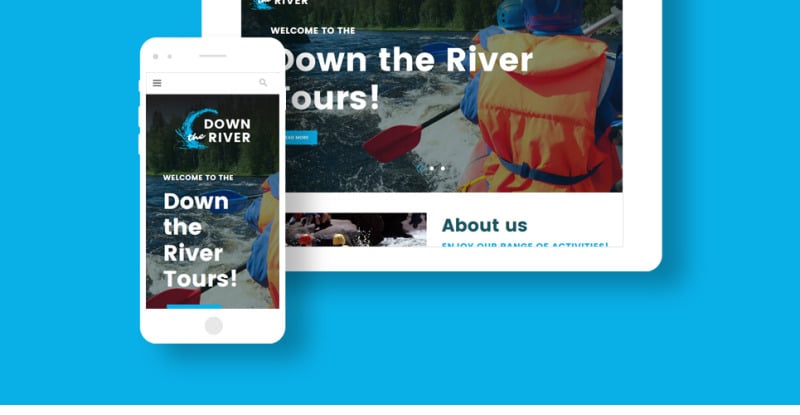The image appears to be a cropped screenshot of an online advertisement, possibly for a travel or tour company, displayed on a computer screen. The background of the image is medium blue, providing a contrasting canvas for the central visual elements. 

In the center, there is a depiction of a tablet showcasing an advertisement with the prominent text "Welcome to Down the River Tours" in white. Adjacent to this text, on the right side of the tablet screen, are two individuals wearing helmets and life jackets, actively paddling a canoe through a river, likely featuring in a whitewater rafting scenario. 

On the left side, below the word "Tours," is a blue clickable button. Unfortunately, the text on this button is indiscernible. Just beneath this button, there's legible text reading "About Us," but anything below is cut off from view.

Overlaying the bottom left corner of the tablet image is a stylized representation of a phone screen. This phone screen displays "Down the River" at the top, followed by "Down the River Tours," mirroring the tablet content. Although the phone screen shows the same rafting image, it is significantly cropped, revealing only a portion of the whitewater and a glimpse of the paddles along with the left arms of the paddlers, whose gender is indeterminate.

The composition of the image effectively highlights the advertising content on both tablet and phone screens, emphasizing the adventure and excitement of "Down the River Tours."